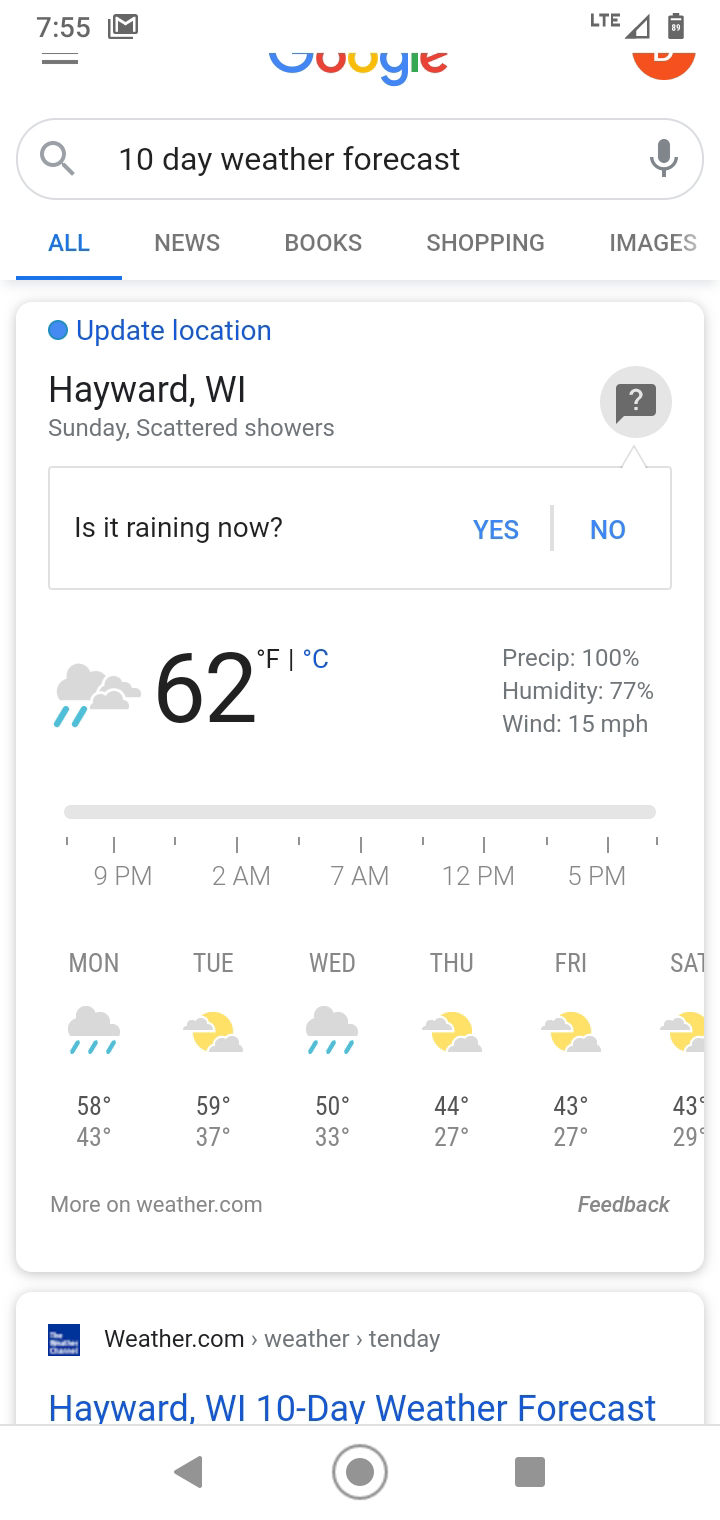**Detailed Caption:**

This image is a screenshot of a smartphone displaying a 10-day weather forecast search. In the top left corner, the time reads 7:55, alongside a Google Mail icon. Next to it, cellular service indicators show LTE, and the internet connection and battery charge icons are visible. The top middle displays the upper portion of the Google logo, while on the right side, there’s a partially visible circular icon. Below, a search bar contains the entry "10 day weather forecast," followed by category tabs labeled All, News, Books, Shopping, and Images, with the All tab highlighted.

Beneath these tabs, a large rectangular box prompts the user to "Update location" in blue font with a nearby blue dot icon. It displays the current location as "Hayward, WI" (Wisconsin). The forecast for Sunday predicts scattered showers, indicated just above a white box bordered by a gray line, which asks, "Is it raining now?" with blue "Yes" and "No" options beside a question mark icon.

Below this, an icon of clouds with light rain appears next to "62°F," followed by a link to switch to "°C." To the right, additional weather details note 100% precipitation, 77% humidity, and winds at 15 mph. A gray bar beneath these details displays time markers from 9 p.m., 2 a.m., 7 a.m., 12 p.m., and 5 p.m.

Subsequently, abbreviations for the days Monday through Saturday are listed, each accompanied by weather icons showing a progression of conditions: rain cloud on Monday, sun with clouds on Tuesday, rain with cloud on Wednesday, cloud with rain on Thursday, and sun with clouds on Friday and Saturday. Below each day, temperature highs and lows are specified: Monday at 58°F/43°F, Tuesday at 59°F/37°F, and Wednesday at 50°F/33°F, with further temperatures continuing in a similar pattern.

At the bottom, there’s a link to "more on weather.com" and an option for feedback. The next box of results features a result for weather.com with its icon on the left.